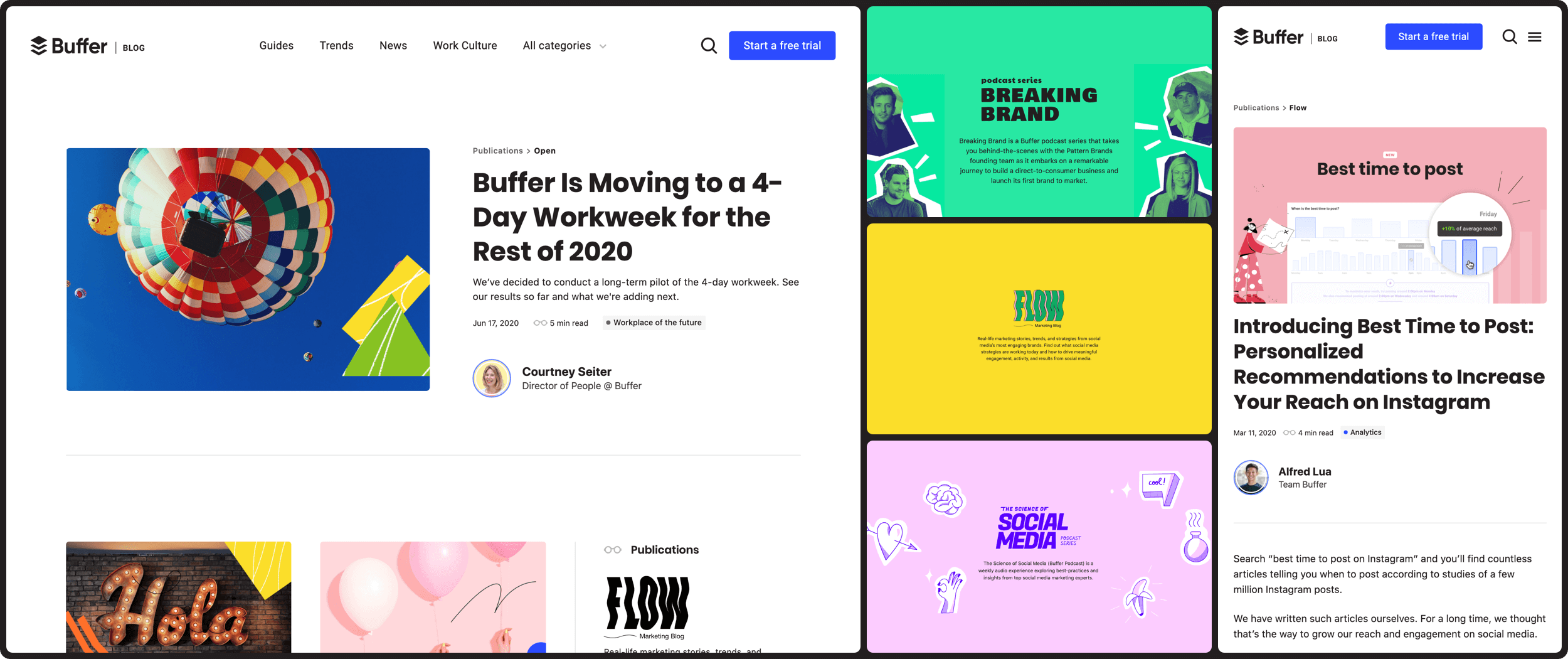**BufferBlog Website Screenshot Description**

This screenshot captures the homepage of the BufferBlog website. At the top of the page, several navigation tabs are visible, including "Guides," "Trends," "News," and "Work Culture," along with an "All Categories" drop-down menu. To the right, there is a blue button labeled “Start a Free Trial,” accompanied by a magnifying glass icon, which presumably represents the search function.

The main content area highlights various articles and features:

1. **Feature Article:**
   - **Title:** "Buffer is moving to a four-day workweek for the rest of 2020"
   - **Summary:** The article announces Buffer’s decision to conduct a long-term pilot of a four-day workweek, including initial results and future plans.
   - **Date:** June 17, 2020
   - **Read Time:** Approximately 5 minutes
   - **Category:** Workplace of the Future
   - **Author:** Courtney Seiter, Director of People at Buffer
   - Accompanying the article's summary are several graphic images.

2. **Podcast Series:**
   - **Title:** "Breaking Brand"
   - **Description:** This Buffer podcast series provides an inside look at the Pattern Brands founding team’s journey in building a direct-to-consumer business and launching their first brand.
   
3. **Flow: Real-Life Marketing Stories, Trends, and Strategies:**
   - **Summary:** This section features stories and strategies from the most engaging brands on social media, offering insights on effective social media strategies and how to drive meaningful engagement and results.

4. **The Science of Social Media Podcast Series:**
   - **Description:** A weekly podcast by Buffer that delves into best practices and insights from leading social media marketing experts.

On the right sidebar:
- **Title:** "Best Time to Post"
- **Summary:** Announcing the introduction of personalized recommendations for the best times to post on Instagram to maximize reach.
- **Date:** March 11, 2020
- **Read Time:** Approximately 4 minutes
- **Author:** Alfred Lua, from Team Buffer
- The summary emphasizes that while many articles suggest optimal posting times based on studies of Instagram post data, Buffer aims to provide personalized insights to enhance social media engagement.

Overall, this screenshot provides a comprehensive look at BufferBlog’s diverse content offerings, ranging from workplace culture insights to social media marketing strategies and podcast series.